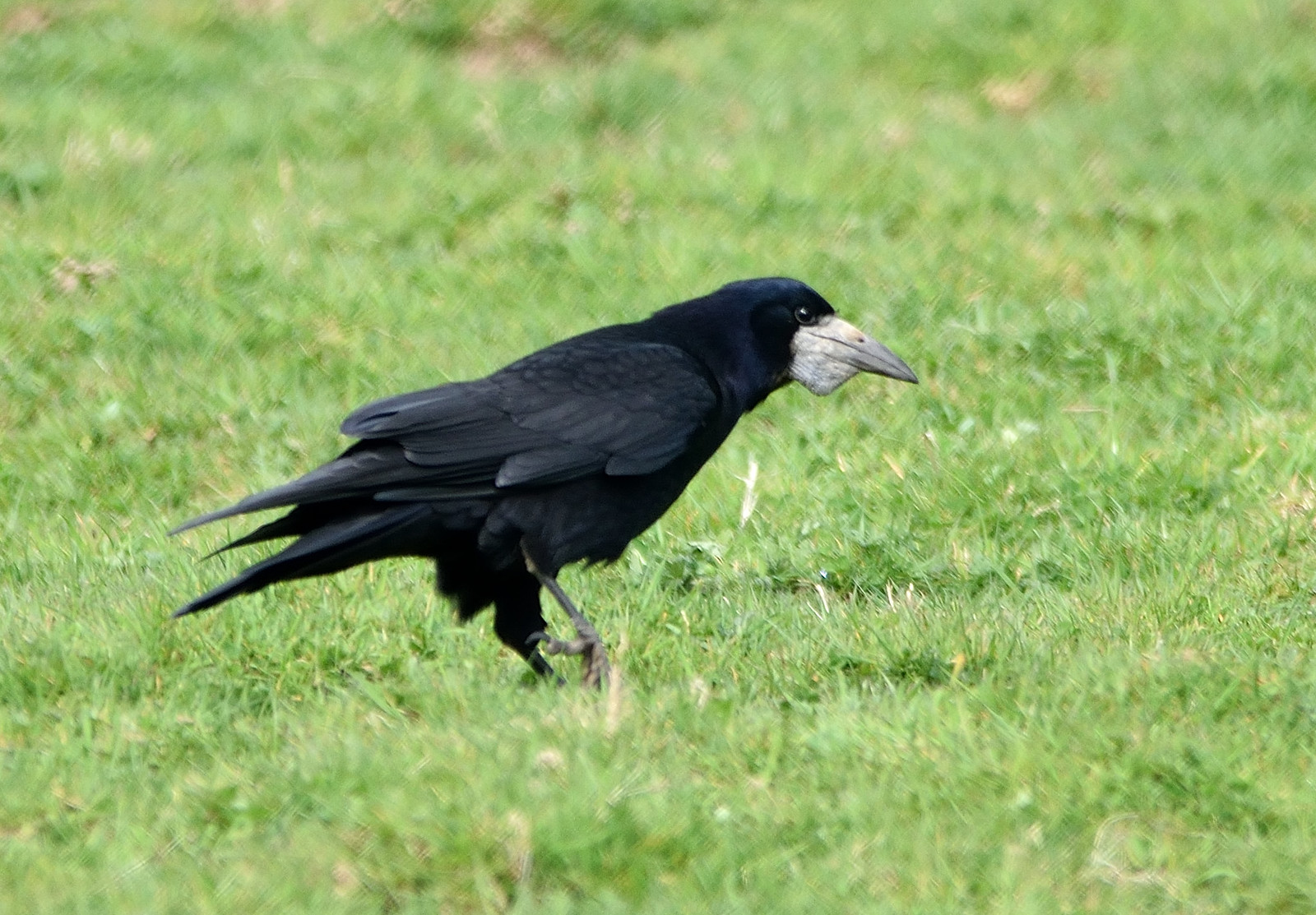A medium-sized black bird, possibly a blackbird or crow, stands with one leg lifted, appearing to take a step in a grassy area filled with tall grass and weeds. The bird has a striking combination of dark black feathers and a gray beak, which transitions from a medium gray at the tip to a lighter gray towards the base, almost appearing off-white. Notably, there's a small, square-shaped protrusion underneath the beak, suggesting some form of growth or perhaps something caught. The bird's white eyes are intently staring into the distance, giving it an angry or determined look. The feathers on its wings show a slight variation in black tones, but the bird remains predominantly dark. It is well-defined against the green background, and there are no visible insects or other distractions around, making the bird the clear focal point of the image.